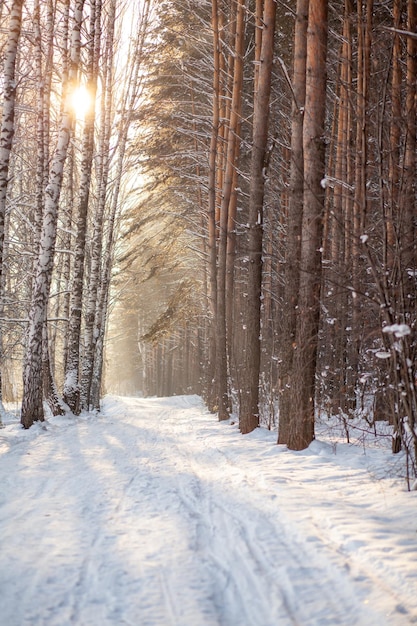The picture captures a bright, sunny winter landscape with a snow-covered road or pathway. There are noticeable old tracks in the snow, likely from a car, but no fresh ones. Tall, slender trees line the path, with their trunks prominently visible. On the left side, the trees have white bark with brown patches, and on the right, the trees have darker brown bark. The sun is high in the sky, casting a glowing reflection onto the glistening snow and adding a serene quality to the scene. In the distance, bare branches cross over the pathway. The ground is blanketed in thick snow, and some far-off trees still have leaves, creating a beautiful contrast against the mostly bare branches closer to the viewer.